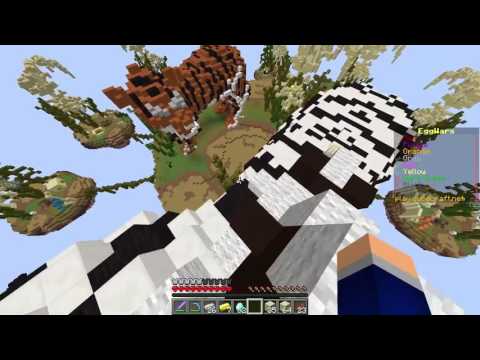A highly detailed and vibrant still shot from the Minecraft video game, the rectangular image is framed by narrow black bars along the top and bottom. In the scene, a character's rectangular block hand, clad in a gray and blue shirt, extends from the lower right corner. The character stands on a large stairway-like structure made from black and white Lego-like blocks, which stretches from the lower left to the upper right corner. This structure curves upwards and seems to hover over a varied landscape set against a light blue sky.

To the left of the stairway, a landform with blocky, splotchy green and brown camouflage-like textures resembling floating islands are visible. One of these landforms features a large brown cow statue prominently placed on it. Additional floating platforms with trees are radially connected around the central cow island, adding depth to the landscape.

At the bottom center of the image, a menu bar displays inventory slots and a health bar depicted with red hearts on the left and a weapon icon, possibly a knife or hammer, on the right. The overall composition hints at the player’s perspective, suggesting exploration within a fantastical Minecraft world teeming with interconnected floating islands and curious structures.